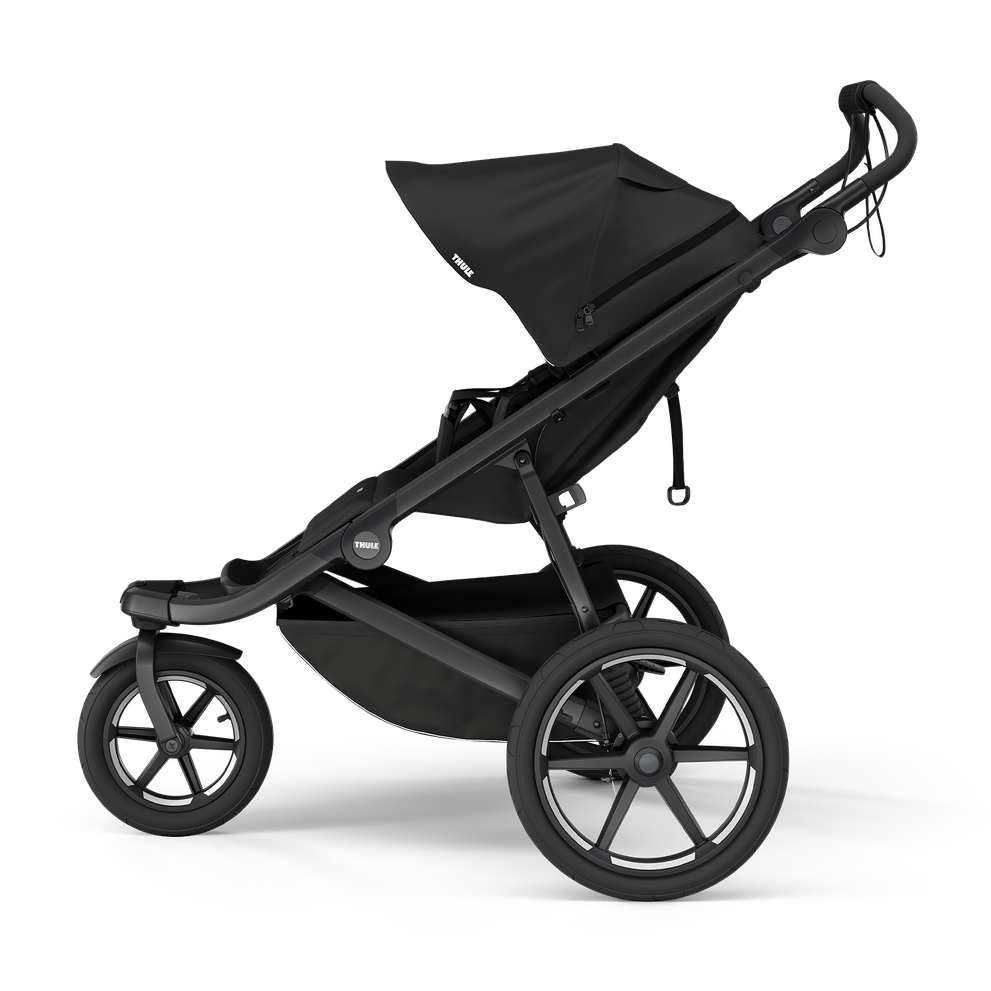This photograph depicts a sleek, black THULE baby stroller set against a plain white background, likely intended for e-commerce display. The stroller features a robust three-wheel design with a smaller, guard-protected front wheel and two larger rear wheels, each wheel displaying six spokes. The tires appear to be inflatable. A black fabric canopy provides shade for the baby, complemented by extendable handlebars that also serve as structural supports. The stroller includes a zipper compartment and a small fabric storage tray situated between the front and rear wheels, adding practical storage options. The overall form is highlighted by a subtle drop shadow beneath, accentuating the tricycle-like wheel arrangement and the diagonal bar that secures the seating area.